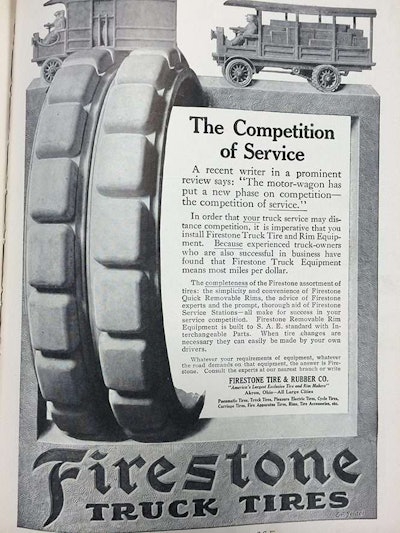This detailed magazine advertisement for Firestone truck tires features a retro aesthetic, primarily in black and white with a grayish stone block dominating the center. The focal point is a large, meticulously detailed illustration of a truck tire showcasing deep treads, which is partially embedded in the stone block. Above this, at the top of the advertisement, are two vintage truck images: a panel truck on the left and an older van-like truck on the right, the latter laden with wooden planks. In the upper right corner, there’s another truck image, indicative of the 1920s or 1930s era, characterized by its open cab design with a vertical steering wheel. Below the tire illustration, the bold slogan "The Competition of Service" is prominently displayed, followed by a detailed write-up describing how motor wagons have revolutionized competitive service. The text consists of several paragraphs, although the bottom ones are quite small and hard to discern. At the bottom of the advertisement, "Firestone Truck Tires" is written in a stylized font with "Firestone" in a slightly fancy script and "Truck Tires" in all capital plain text, reinforcing the advertisement’s focus.